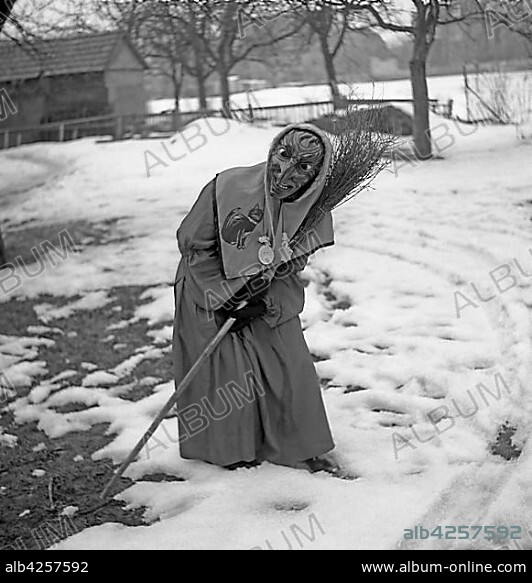In this black and white photograph, a mysterious figure dressed as a witch stands in a snow-covered field. The person is cloaked in a gray robe and wears gloves, with a hood covering their head adorned with a small black cat. They also don an eerie mask. The figure holds a traditional broomstick in their right hand. The landscape reveals bare trees stretching across the entire image, suggesting a cold winter's day. In the background, to the left, sits a gray-colored cabin, accompanied by a fence and a car. The scene is devoid of any animals, emphasizing the barren, wintry setting. Across the top of the image are branches and stems without leaves, intensifying the desolate atmosphere. At the bottom of the photograph, the text "ALB4257592" appears twice in gray against a black strip, along with the website "www.album-online.com" in white.